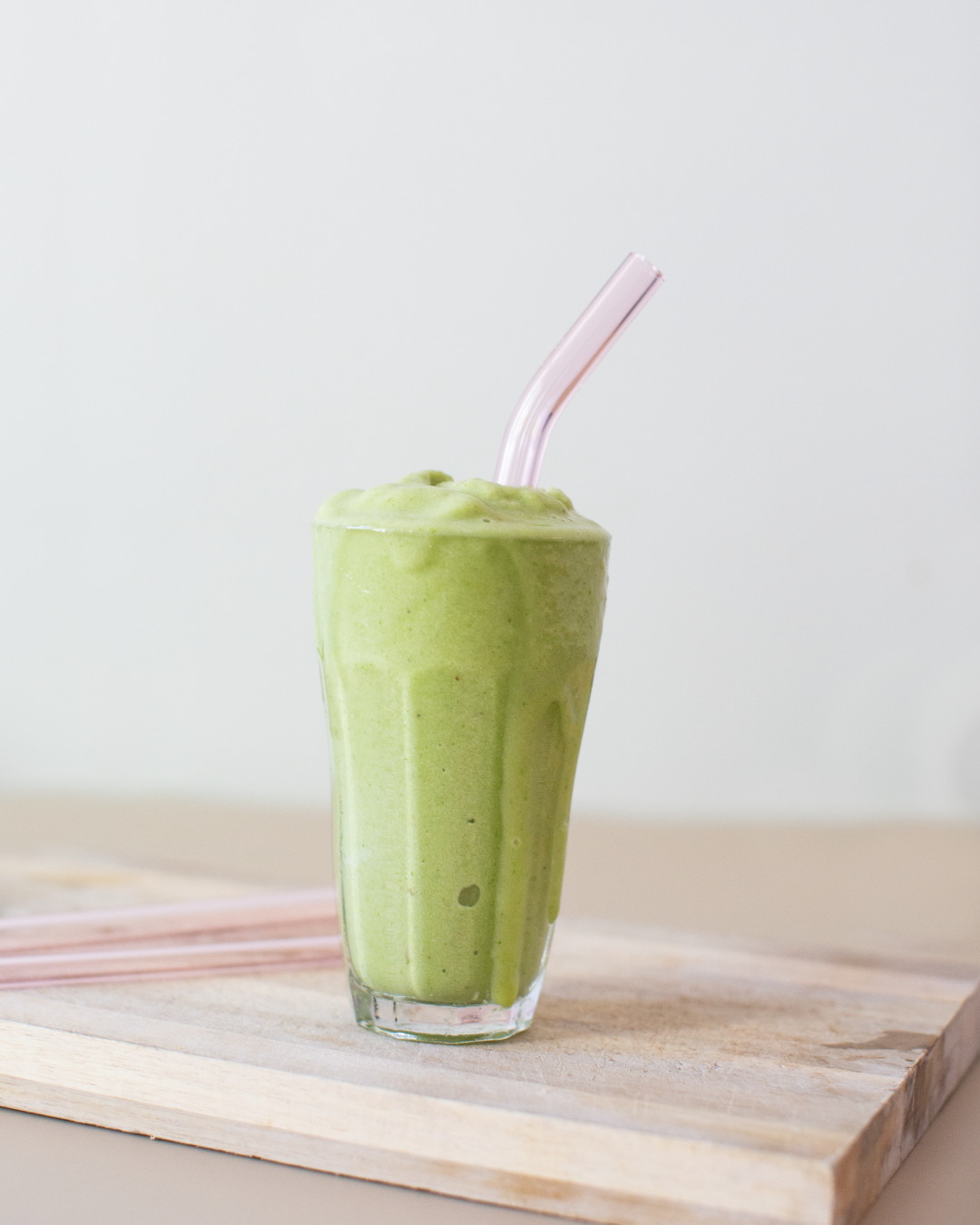The image depicts a tall, clear crystal glass filled to the brim with a thick green liquid that could be a green smoothie or milkshake, potentially made from avocado, green tea, or a mix of various green ingredients. The consistency appears creamy and is overflowing slightly, with small bubbles visible in the liquid. A prominent, clear pink straw sticks out from the top, and two additional pink straws lie on a beige and brown butcher block placed on a light beige wood table. The background features a white wall, and the scene conveys a sense of indulgence and freshness.